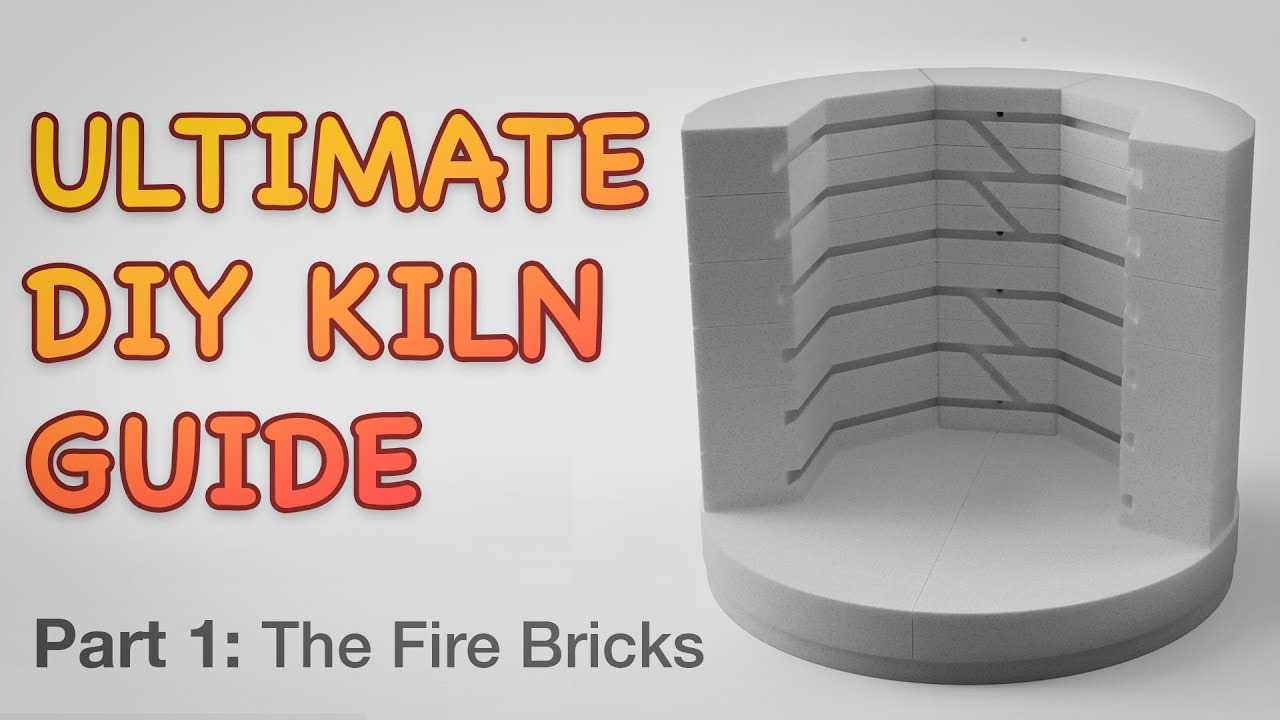This image, resembling a photo from a book or brochure, is an advertisement for the "Ultimate DIY Kiln Guide, Part 1: The Fire Bricks." The advertisement is a horizontally oriented rectangle with a clean, white background. On the left side, the title is prominently displayed in large, gradated gold-to-red bubble lettering, with "Part 1: The Fire Bricks" written in black underneath it. The right side of the image features a detailed cross-section of a kiln, constructed from interlocking, gray fire bricks and resting on a gray base. The kiln's cutaway design reveals six internal levels, though intricate details about its functionality remain obscure. The primary colors are the yellow-to-orange gradient of the title and the various shades of gray in the kiln and its base, creating a stark, monochromatic aesthetic peppered with warm hues from the text.